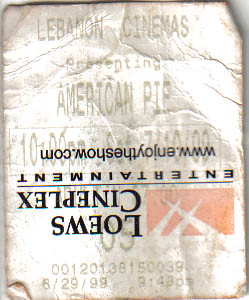The image captures an old, weathered movie ticket stub. Overlayed on the photograph, there is a clear, dark piece of computer-generated text, positioned upside down. This text reads "Lowe's Cineplex Entertainment" in black font, along with the website URL "www.enjoytheshow.com". In the background, the original ticket stub features the heading "Lebanon Cinemas presenting American Pie" in a faded black font. Below this, the stub displays the screening time and a red logo situated in the lower right corner. At the very bottom, in less visible text, the date and time are marked as June 29th, 1999 at 9:48 PM. The edges of the ticket stub show signs of age, with bent, dog-eared, and frayed corners, adding to its vintage appearance.